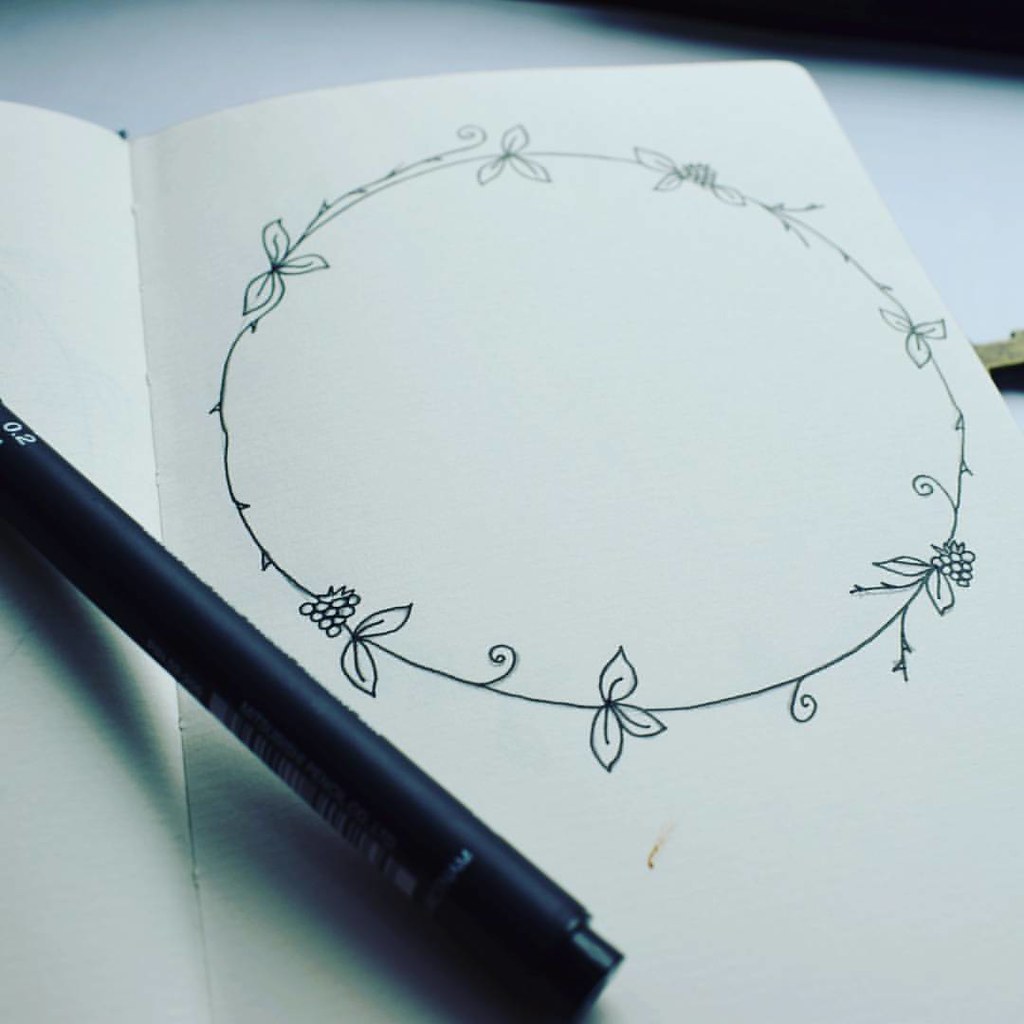The photograph showcases a detailed, hand-drawn sketch in a notebook. The camera angle is nearly parallel to the page, immersively capturing the fine details of the drawing and the notebook itself. The sketch, rendered in black pen, features a circular design surrounded by intricate thorns, giving the impression of a thorny wreath. Interspersed within the thorns are clusters of two to three leaves, distributed evenly every few inches. Additionally, the design includes elements resembling the number nine, though each 'nine' features an extended curl, deviating from the usual shape. A thick black pen or pencil, marked with "0.2" in white lettering, rests on the edge of the notebook. The paper of the notebook is distinctly white and appears to be of a higher thickness, providing a sturdy backdrop for the artistic sketch.